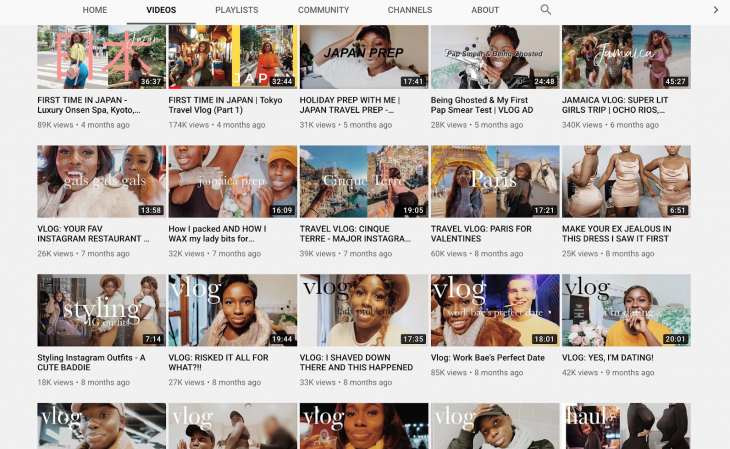The webpage appears to be a vlog channel, displaying a collection of various video content. The navigation bar at the top includes tabs labeled "Home," "Videos," "Playlists," "Community," "Channels," and "About." The current section shown is the "Videos" tab, revealing a grid layout consisting of five columns and four rows of video thumbnails.

The video titles, listed in order, are as follows:
1. "First Time in Japan - Tokyo Travel Vlog"
2. "Luxury Onsen Spa Holiday - Prep with Me"
3. "Japan Travel Prep: Being Ghosted and My First Pap Smear"
4. "Super Lit Girls Trip Vlog"
5. "Your Favorite Instagram Restaurant"
6. "How I Packed and How I Wax My Lady Bits - Travel Vlog"
7. "Sneak Peek: Major Instagram Travel Vlog"
8. "Paris for Valentine's: Make Your Ex Jealous in This Dress"
9. "I Saw It First: Styling Instagram Outfits"
10. "A Cute Baddie Vlog"
11. "Risked It All for What? - Vlog"
12. "I Shaved Down There and This Happened - Vlog"
13. "Work Base: Perfect Date Vlog"
14. "Yes, I'm Dating!"

The final row contains additional video thumbnails, but the titles are unfortunately cut off and unreadable. The overall page is densely packed with an array of engaging and diverse vlog videos, each offering a glimpse into different aspects of the vlogger's life and travel experiences.